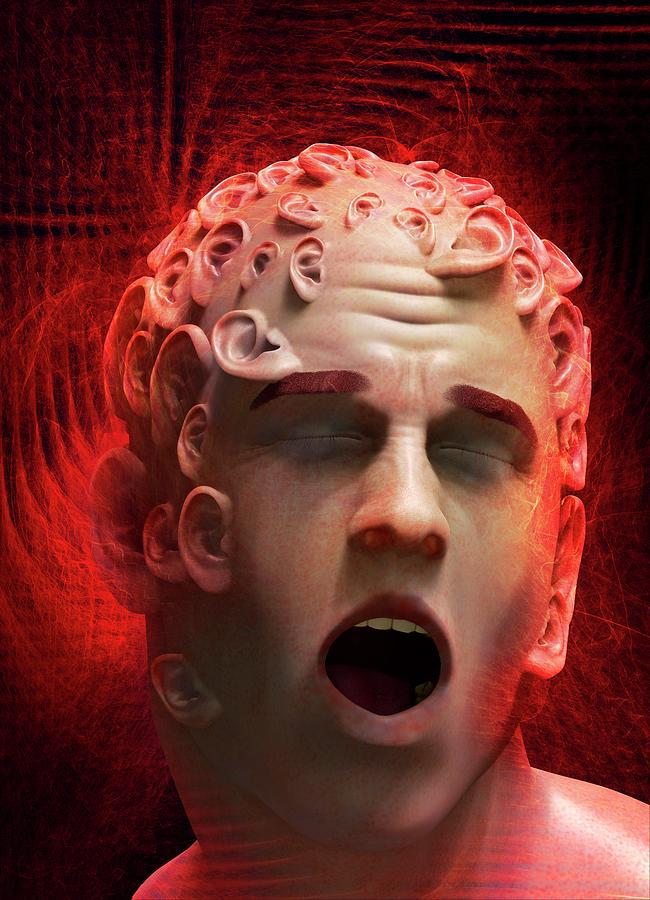In this intriguing and somewhat haunting artwork, we see a man depicted against a predominantly reddish, holographic background accented with black and red echoes. The man's face, painted in shades of black, red, and tan, presents a striking anatomical anomaly: his head is entirely covered by numerous ears of various sizes, including two particularly large ones in the background. These ears extend from the sides of his head down to his cheeks, replacing where hair would typically be. The man’s eyes are closed, and his mouth is open, exposing his top row of white teeth, leaving viewers uncertain whether he is experiencing agony or ecstasy. The man's thick, bushy brown eyebrows and a few wrinkles on his forehead add to the depth of the expression. The detailed, almost carved-out appearance of his face and ears, combined with the eerie background, creates a surreal and mesmerizing visual impact.